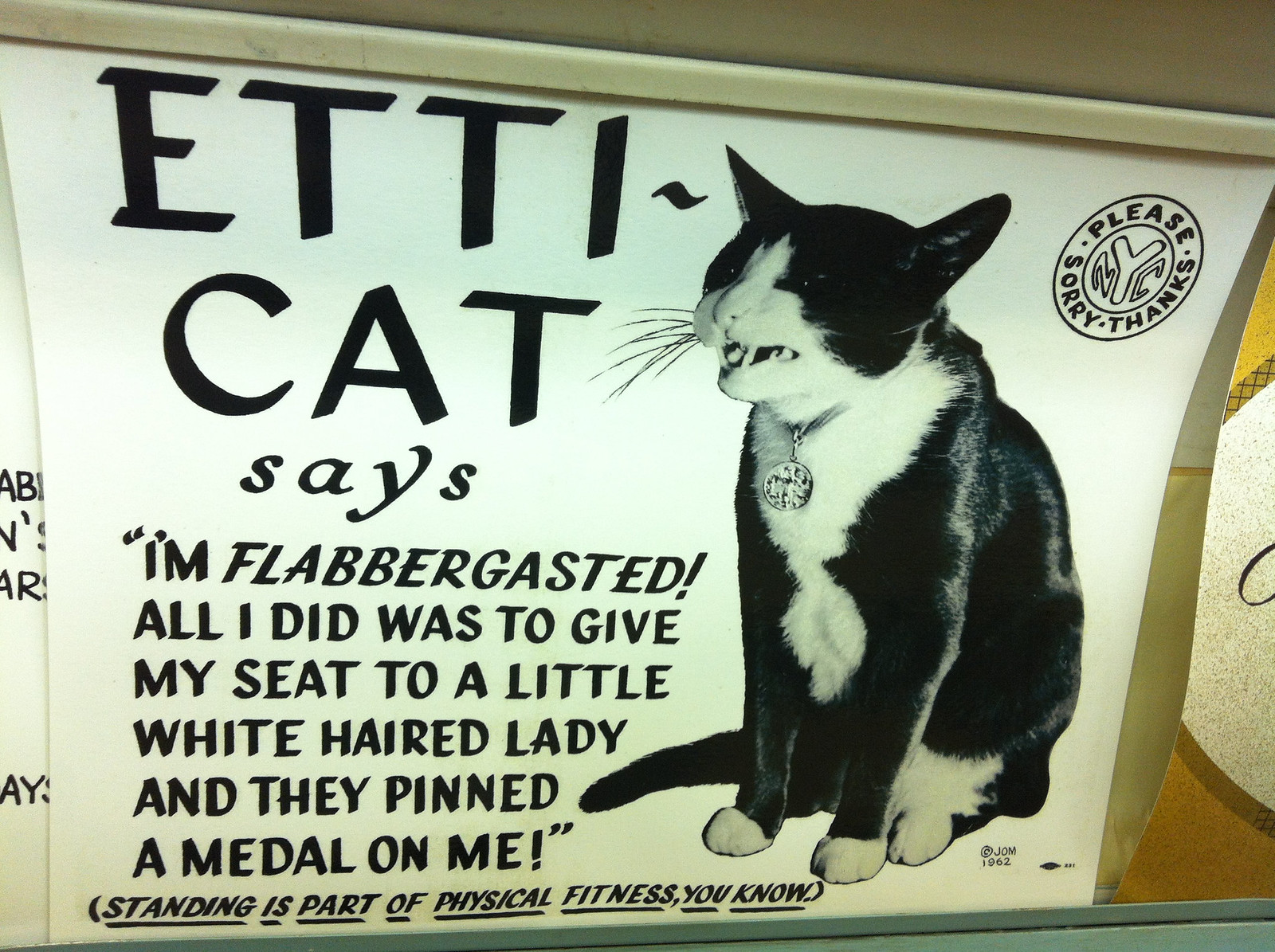The image is a subway advertisement poster featuring an anthropomorphized black and white cat named Eddie Cat. Eddie Cat, adorned with a collar that has something hanging from it, is depicted with long whiskers, teeth showing, and ears erect, giving an impression of readiness to bite. Alongside the cat, there is text in black letters against a white background. On the left side, it reads: "Eddie Cat says, I'm flabbergasted! All I did was to give my seat to a little white-haired lady and they pinned a medal on me. Standing is part of physical fitness, you know." On the right side, there is a circular badge with the words "please, sorry, thanks" encircling the letters "NYC." Below the cat is some small, unreadable text. The overall setup is reminiscent of the advertisements typically seen above the seats inside New York City subway cars, lit from behind for visibility.